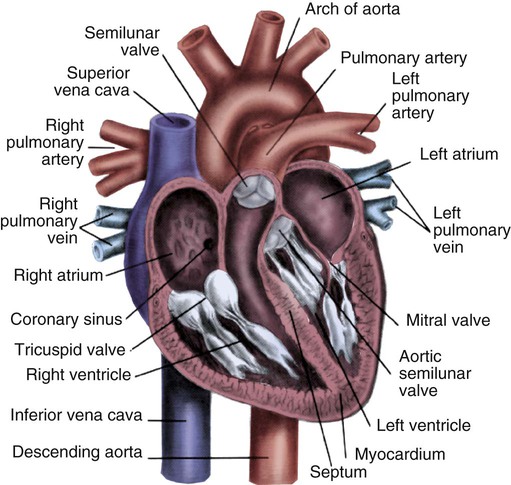This vertical image, reminiscent of an illustration from a science textbook, intricately depicts a detailed drawing of a human heart in a cross-section, presenting an x-ray-like view to reveal the inner workings. The heart is delicately sliced to show all the chambers, valves, and major blood vessels: veins, arteries, ventricles, and more—all meticulously labeled.

At the top, the arch of the aorta, characterized by three tubes extending from a rounded section, is prominently displayed. To the left, the superior vena cava, depicted in blue, resembles a pipe, while the right pulmonary artery appears as three finger-like projections. Below these, the right pulmonary vein, also blue, is similar in structure to the arteries.

Central to the diagram, the heart's interior reveals two semicircles—the right atrium on the left, marked in red, and the left atrium on the viewer's right. Directly below, the left pulmonary vein is depicted as two small tubes emerging from the atrium's smooth section. Surrounding the central chambers are the white, ghost-like tricuspid and mitral valves, along with the aortic semilunar valve, all distinctly highlighted.

Color-coded for clarity, everything related to veins is illustrated in blue, while arteries are in red, with steel blue, white, and shades of maroon accentuating various parts. Blood vessels leaving the top of the heart and other key components like the myocardium—a lining around the heart—and the septum, which separates the heart's parts, are also indicated. At the bottom, two tubes represent the inferior vena cava and the descending aorta, with the former in blue and the latter in red. The detailed nature and thorough labeling of this diagram provide a comprehensive view of the cardiovascular system.